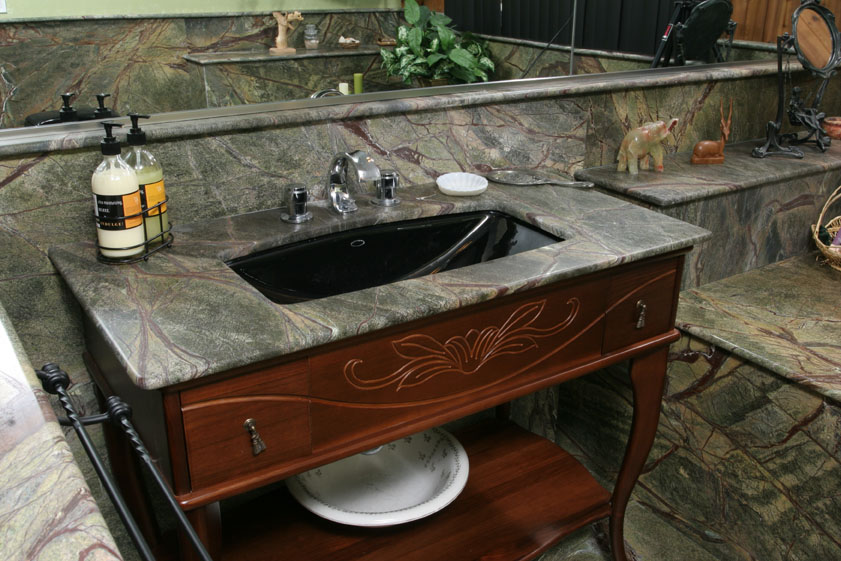This image is a color photograph showcasing an exquisitely designed luxury bathroom, possibly within a high-end hotel or an opulent private residence. The ambient lighting highlights the elegance of the space. Dominating the foreground is a sleek wooden vanity, topped with a striated marble or stone countertop that seamlessly extends up the backsplash. The countertop features a sophisticated black basin sink, contrasting beautifully with the countertop.

On the countertop, beside the sink, sits a bar of soap, adding a practical touch to the decor. Below the sink, the vanity includes a drawer, which might be a faux drawer, adding to the streamlined design. Underneath this drawer, a shelf holds a pristine white porcelain bowl, further accentuating the luxurious yet functional nature of the space.

The right side of the photograph captures a glimpse of a lavish bathtub, which is partially obscured but suggested by the elaborate stone wall that surrounds the bathroom. This wall ties the entire room together, giving it a cohesive and indulgent feel.

Adorning the area above the bathtub, a jade elephant, a wooden deer figurine, and various other decorative accessories occupy a shelf, imparting a personalized and exotic touch to the room. The bottom edge of this shelf holds a basket, partially visible, adding an element of storage or decor.

A large mirror runs along the top edge of the image, reflecting parts of the background and enhancing the room's spaciousness. Reflected in the mirror, a plant and several other objects hint at the viewer's surroundings, completing the scene with an inviting and lived-in ambiance.